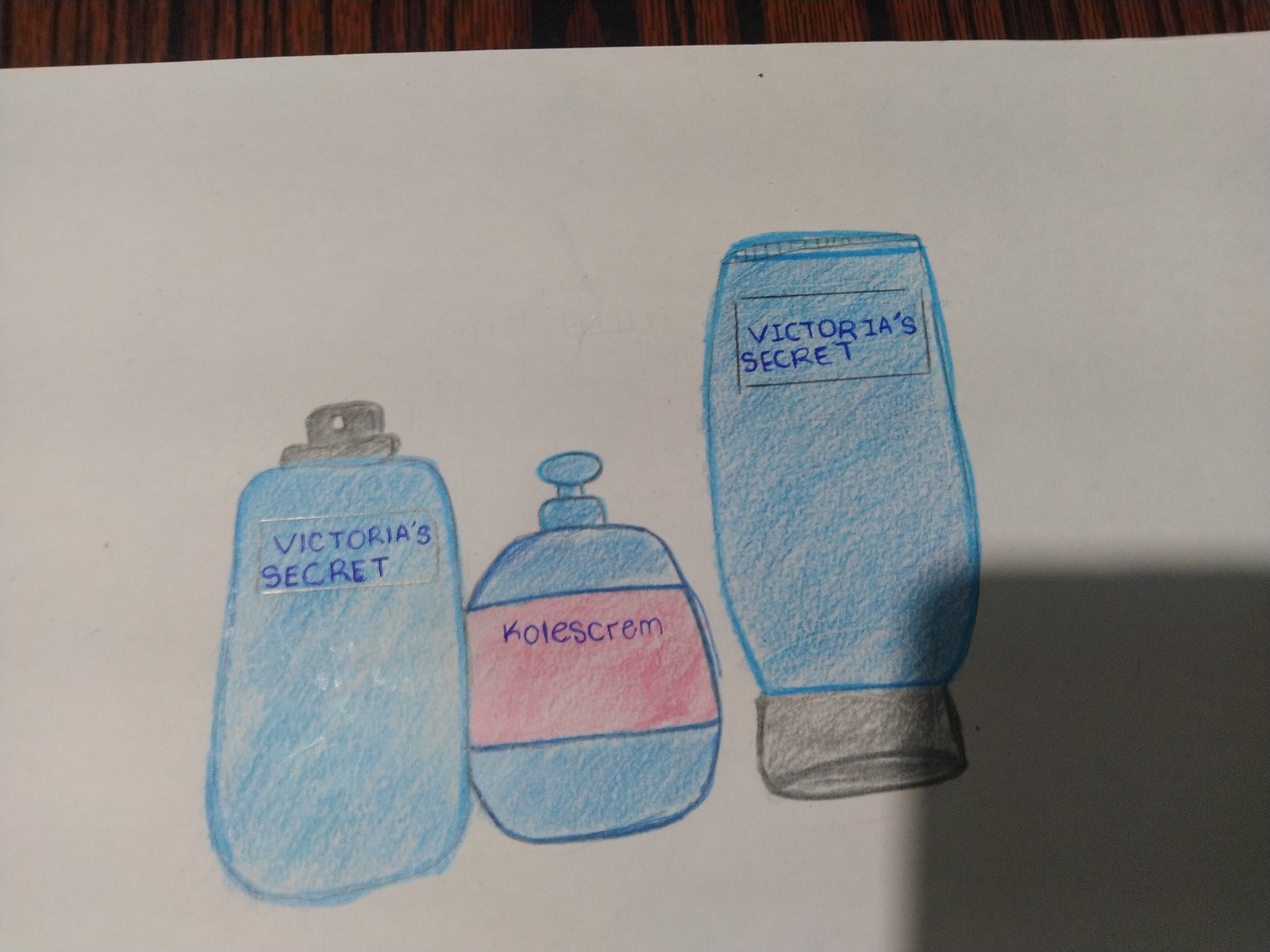This color photograph captures a detailed pencil or crayon drawing on a large sheet of white drawing paper. Central to the artwork are three distinct objects: two bottles and a small soap dispenser. To the left, a rectangular Victoria's Secret bottle is shaded in light blue and is topped with a gray cap. "Victoria's Secret" is inscribed in blue ballpoint pen on this bottle. Slightly behind and next to it is a small soap dispenser bottle, marked "K-O-L-E-S-C-R-E-M" on a pink strip. This bottle is also shaded in blue, with its dispenser rendered in the same color. The largest item, positioned to the right, resembles a Victoria's Secret cream bottle. Shaded in blue, it has an inscription of "Victoria's Secret" at the top. The bottle's dark gray cap rests on the table at the bottom of the image. A square shadow overlaps part of this bottle, encroaching from the bottom right corner of the drawing.